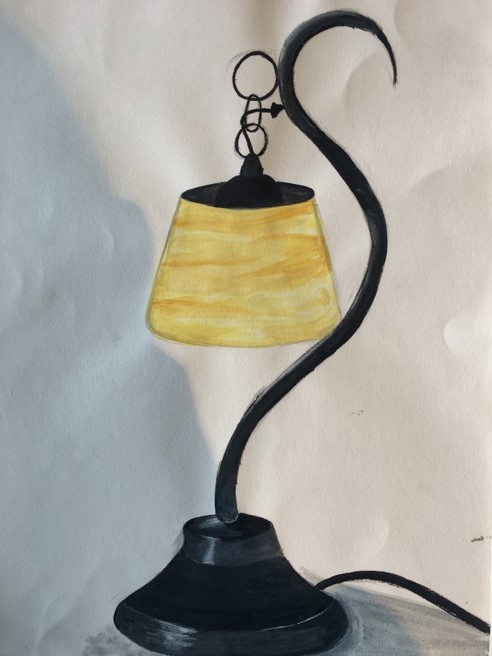The rectangular painting, oriented with its longer side vertical, depicts an elegantly designed end table lamp. The lamp features a black, concave circular base from which a sleek black power cord extends to the right, descending before exiting the frame at the bottom right corner. Rising from the base is a gracefully curved black post, sculpted in a sweeping S-shape that loops back at the top. At the apex of the post, a matching black attachment secures the lamp's shade. The shade emits a warm, golden glow, suggesting the lamp is lit, casting a soft, inviting light that contrasts beautifully with the darker elements of the lamp’s structure.